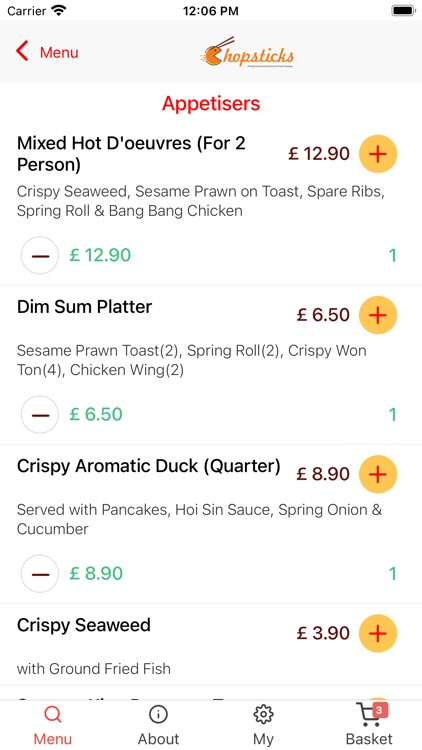**Detailed Caption:**

The image depicts a screenshot of a smartphone displaying a restaurant menu in an app. At the top of the screen, the status bar shows the carrier information, an internet connectivity icon, the time (12:06 PM), and a full battery icon on the right. Immediately below the status bar, there is a light gray navigation bar featuring a red caret pointing left alongside the word "Menu" also in red.

Dominating the central part of the screen is the restaurant name "Chopsticks" rendered in dark yellow cursive. Notably, the 'C' in "Chopsticks" is stylized as a Chinese fortune cookie with chopsticks emerging from the cookie.

The menu title, "Appetizers," is misspelled as "APPETISCRS" in red text. Below this title, four appetizer items are listed:

1. **Mixed Hors D'Oeuvres** - Misspelled as "Mixed Hot D’Oeuvres", it's priced at £12.90. A yellow circle with a plus sign allows adding the item to the order, and a blue circle with a minus sign for decreasing the quantity. The description mentions it is meant for two people and includes crispy seaweed, sesame prawn on toast, spare ribs, spring rolls, and bang bang chicken.

2. **Dim Sum Platter** - Priced at £6.50, with similar plus and minus icons for adjusting the quantity. It includes two sesame prawn toasts, two spring rolls, four crispy wontons, and two chicken wings, as indicated by numerical parentheses.

3. **Crispy Aromatic Duck** - Offered as a quarter portion, priced at £8.90, with the same increment and decrement icons for quantity control.

4. **Crispy Seaweed** - Priced at £3.90, also featuring the standard plus and minus quantity controls.

At the bottom of the screen, there are navigation options: "Menu," "About," "My" (likely referring to account or orders), and "Basket," with "Menu" being highlighted, indicating that this section is currently being viewed.